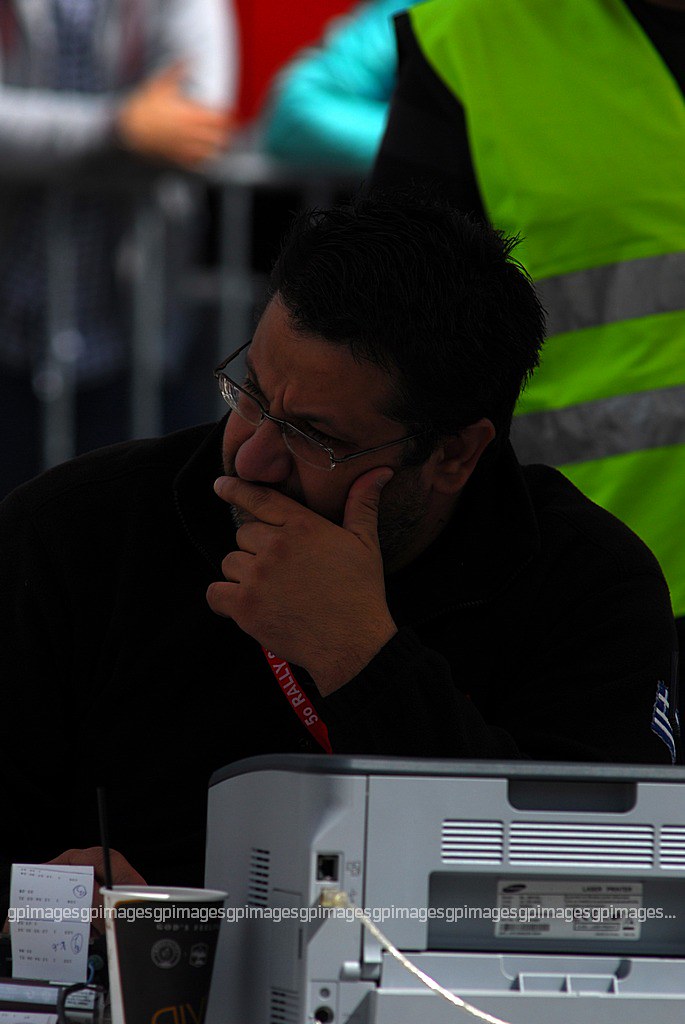The photograph depicts a thoughtful and concerned-looking man seated behind a desk or table. He is visible from the lower chest to the top of his head. The man has short black hair, a stubbly beard, and is wearing small black-framed glasses. He is dressed in a long-sleeve, soft-looking black coat with a blue flag on the sleeve. Around his neck, there is a red lanyard with white text that reads "50 Rally." He has his hand up to his mouth, as if in deep thought, and is looking at something off-screen towards the bottom left corner of the image. 

In front of him on the table, there is a square-shaped machine, likely a printer, and a styrofoam cup, suggesting he might be having coffee. Behind the main subject, slightly blurred, stands another person wearing a sleeveless yellow safety vest with reflective silver bands. The photograph also features a watermark running along the bottom, composed of white text that repeats "GP images."